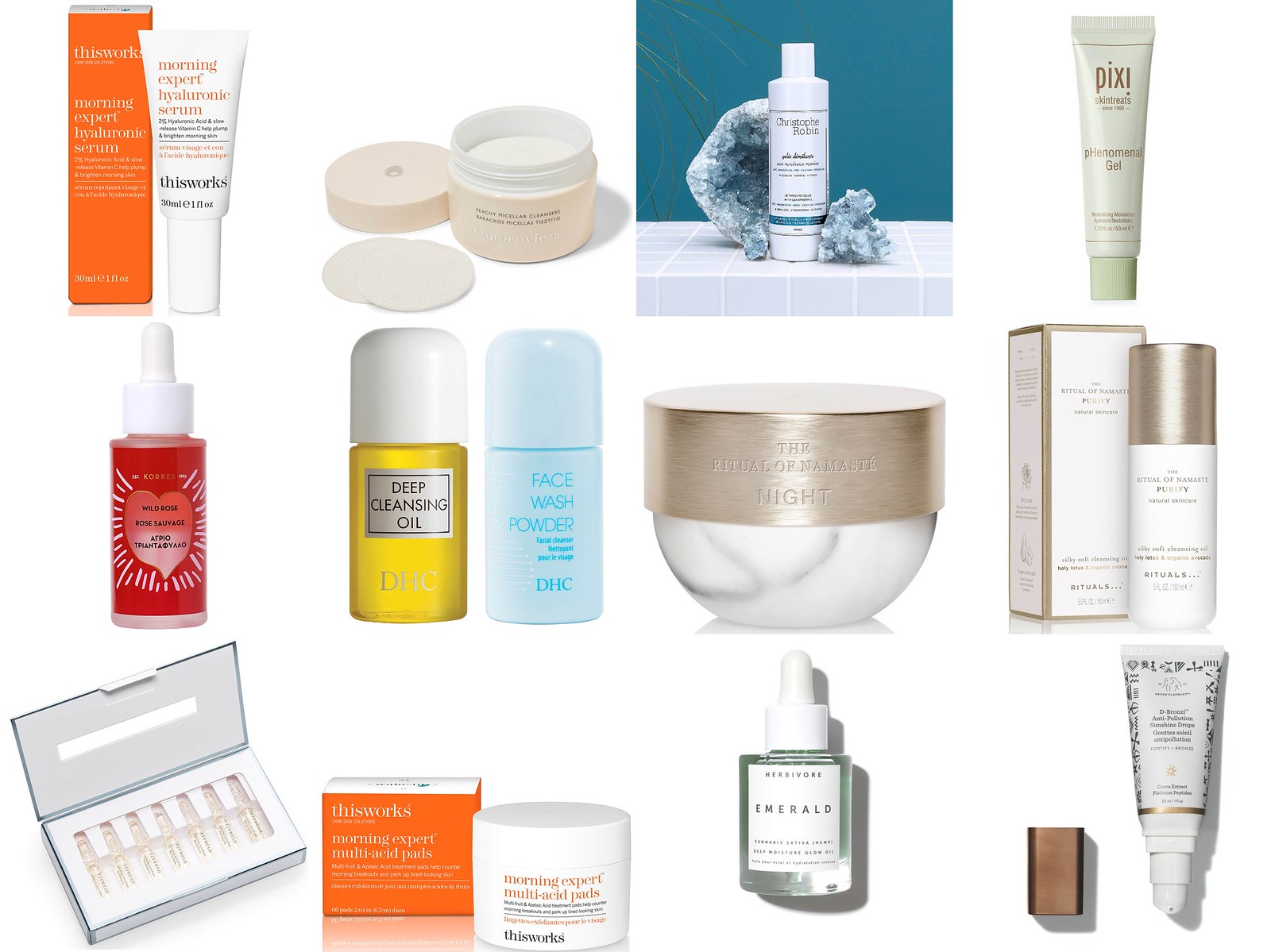The image features a series of individual pictures of various beauty items and toiletries arranged side by side against a featureless white background. The layout is organized into three rows, each containing four items.

**Top Row:**
1. An orange packaging with a separate white tube displayed next to it. The product is identified as "This Works Morning Expert," a hyaluronic serum.
2. A tub with its lid removed, revealing some pads in front of it intended for applying the cream from inside the tub. The writing on the tub is illegible.
3. A tube of "Christoph Robin" product, possibly bath lotion, displayed beside a bath setting with some cloth items that might be used to apply the lotion.
4. A product named "Pixie," which is described on the tube as a pH gel or phenomenal gel.

**Middle Row:**
- Four different products are arranged side by side, but their specific details and descriptions are not provided.

**Bottom Row:**
- Similar to the middle row, four distinct products are displayed in a side-by-side arrangement without specific details.

Each item is presented individually, but the careful editing makes the collection appear as one cohesive image against the plain white backdrop, highlighting the products.